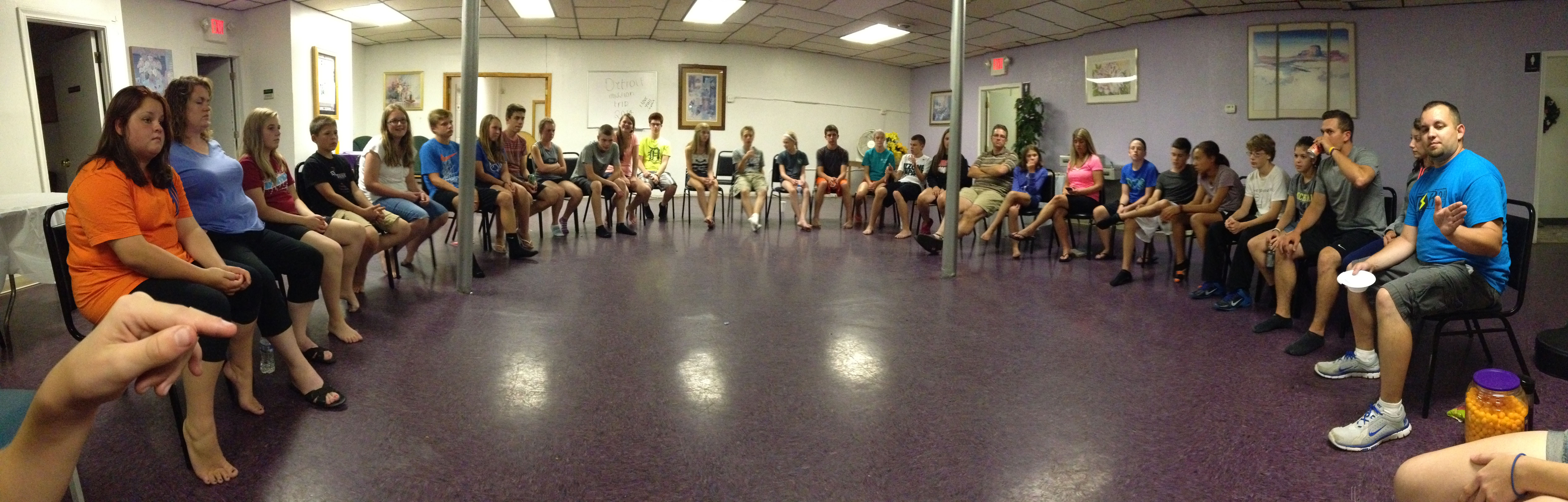This photograph captures an indoor scene of a spacious room with various people seated in a large semi-circle. The room has white walls adorned with artwork, while the wall to the right is a light purple. Prominent support beams stand towards the center of the room, and about 25 to 30 individuals of different ages and genders occupy the chairs arranged in the circle. Some participants wear shoes, while others are either in socks or barefoot. The floor is purple with a speckled pattern, and reflections from the ceiling lights can be seen on it.

In the foreground, on the left side of the image, there is a partially closed hand visible, seemingly gesturing or preparing to pass something. On the right, there's a person's seated legs and another hand. A container of cheese balls is placed on the floor, and one person, who appears to be gesticulating and might be speaking, holds a bowl, possibly to share the cheese balls. An exit sign glows red in the background, emphasizing the room's function as an office or classroom.